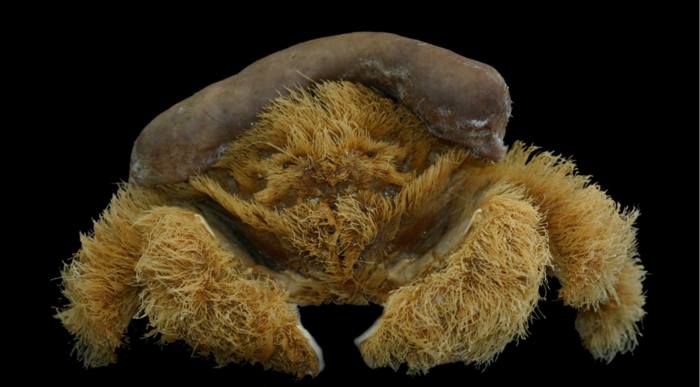The image is a horizontally-oriented photograph, approximately one and a half times wider than it is tall, with a completely black background. In the center of the image is a creature that most closely resembles a crab, though it has the unusual characteristic of being entirely covered in light brown, yellowish fur. This fur obscures its true form, creating a teddy bear-like appearance with four visible legs extending from its body and two curved front claws positioned as if in a defensive or preparatory posture. The creature also features two small, beady eyes at its center. Draped across its back, right behind its head, is a brown, slug-like object, curving in a shape that lies somewhere between a straight line and a "C". The overall effect is that of a peculiar marine organism, possibly a hybrid between a crab and a very furry spider, with an object resembling either a misshaped rock or fish resting atop it.